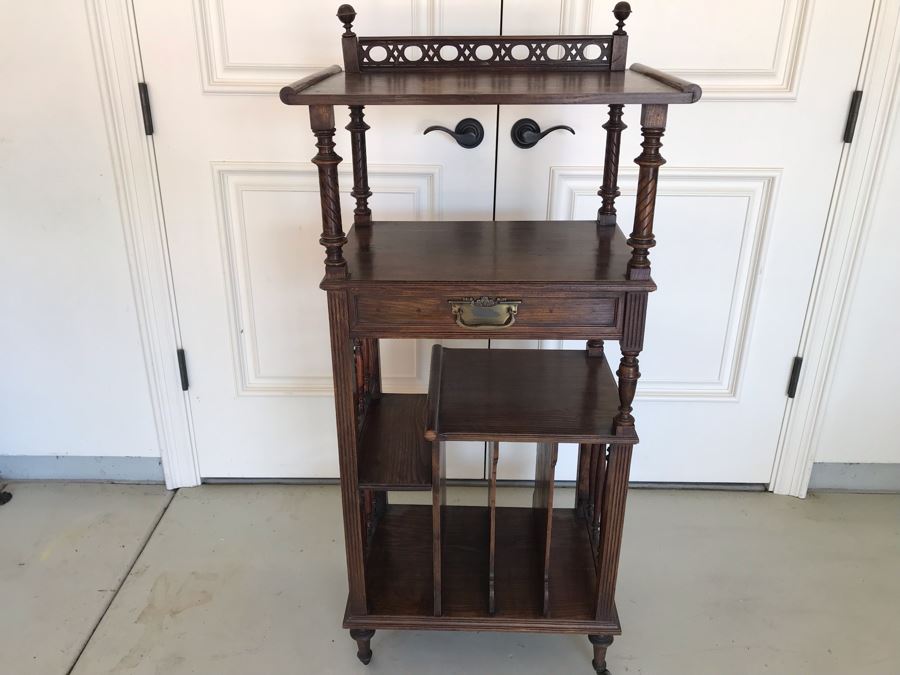This outdoor photograph captures a vintage-style wooden cabinet, beautifully showcased in natural lighting against white walls adorned with double black-handled doors. The cabinet, approximately three feet tall and two feet long, is made from dark walnut-stained wood. It stands on stone pavers. The design features are intricate, including vertical slats at the bottom, apparently tailored for storing magazines or vinyl records. The slats on the left seem to accommodate smaller records, while the three taller slots on the right are suited for standard 12-inch records. Above these, there are two shelves—the lower one being narrower. Sitting between the middle shelf and the top shelf is a single, long, narrow drawer with a bronze handle. This drawer might be used to store keys, wallets, or small trinkets. Elevated above the drawer, the flat top provides additional space, ideal for placing a record player, and is bordered by four wooden columns that reach up to another raised shelf, perfect for showcasing or setting aside other items.